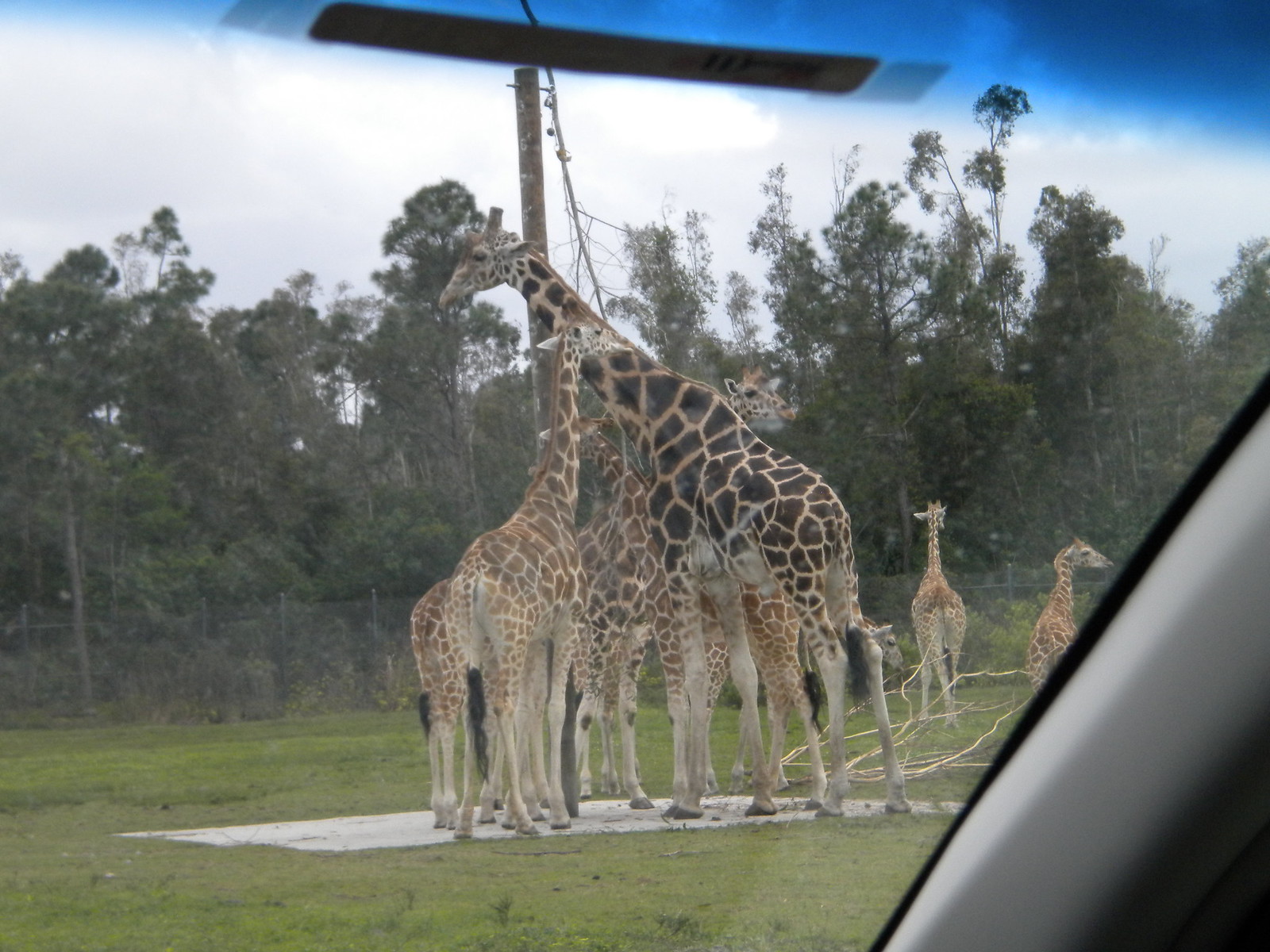A photograph taken through the windshield of a vehicle shows a scene from what appears to be a drive-through safari zoo. The top portion of the image is tinted blue by the translucent sunshade at the top of the windshield, and the right side features a pillar of the vehicle's interior. Beyond the windshield, the open field hosts a group of giraffes standing close together in the center. One notably taller giraffe with darker black spots stands out on the right side, possibly an adult, accompanied by several smaller, juvenile giraffes scattered in the background. There is a hint of chain link fencing with vertical posts at the base of the image, though the details are somewhat obscure. The background rises to tall, dark green trees of varying heights, silhouetted against a heavily clouded sky with light grey and white clouds, creating a lush and moody backdrop for the serene wildlife encounter.